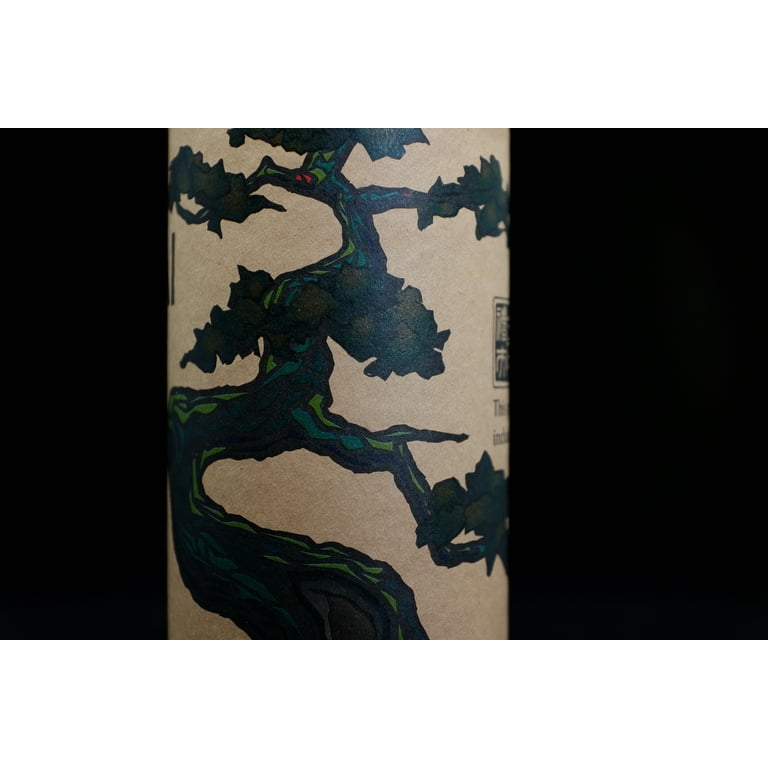The image features a photograph of an abstract piece of art with a black background, occupying around 60% of the frame. Dominating the center, slightly towards the left, is a cylindrical object with a tan backdrop adorned with a unique, winding, and bending tree that stretches upwards. This tree has a striking blue-green color and multiple branches, each adorned with green leaves. The dark, swirling design of the tree gives a somewhat sinister impression. Additionally, small red dots are subtly visible near the top. On the right side of the cylindrical object, partially hidden as if the object is rolled or curved, there is an inscription, although the text remains unreadable.